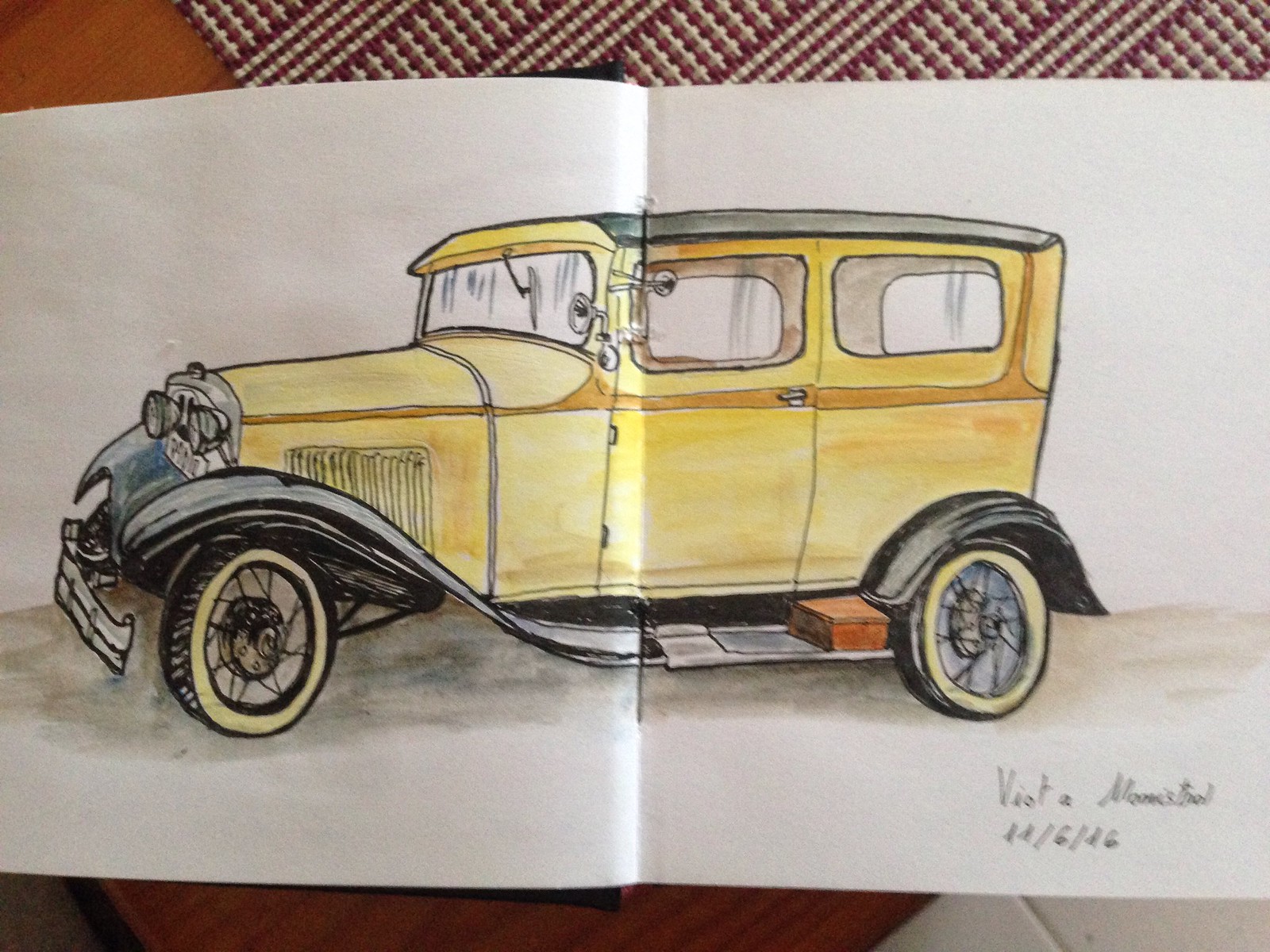In this detailed illustration, presented as a watercolor drawing on an open book lying on a dining table with a placemat behind it, we see an antique, yellow Ford car, evocative of the 1940s. The vehicle stands out with its mostly yellow body contrasted by black fenders and whitewalled tires featuring prominent wire spokes. It boasts a long, rectangular shape with substantial rectangular windows and a flat roof extending straight to the back, where it lacks a traditional trunk. The elongated front showcases a broad hood adorned with radiator grills and crowned by two headlights protruding from a gleaming chrome radiator, accompanied by a substantial chrome bumper. The metal of the car curves gracefully around both the front and rear tires. The artist's signature, although somewhat unclear, appears to read "Miss Vista Marist Roll," and the date "11-6-16" is also inscribed, indicating the time of its creation.